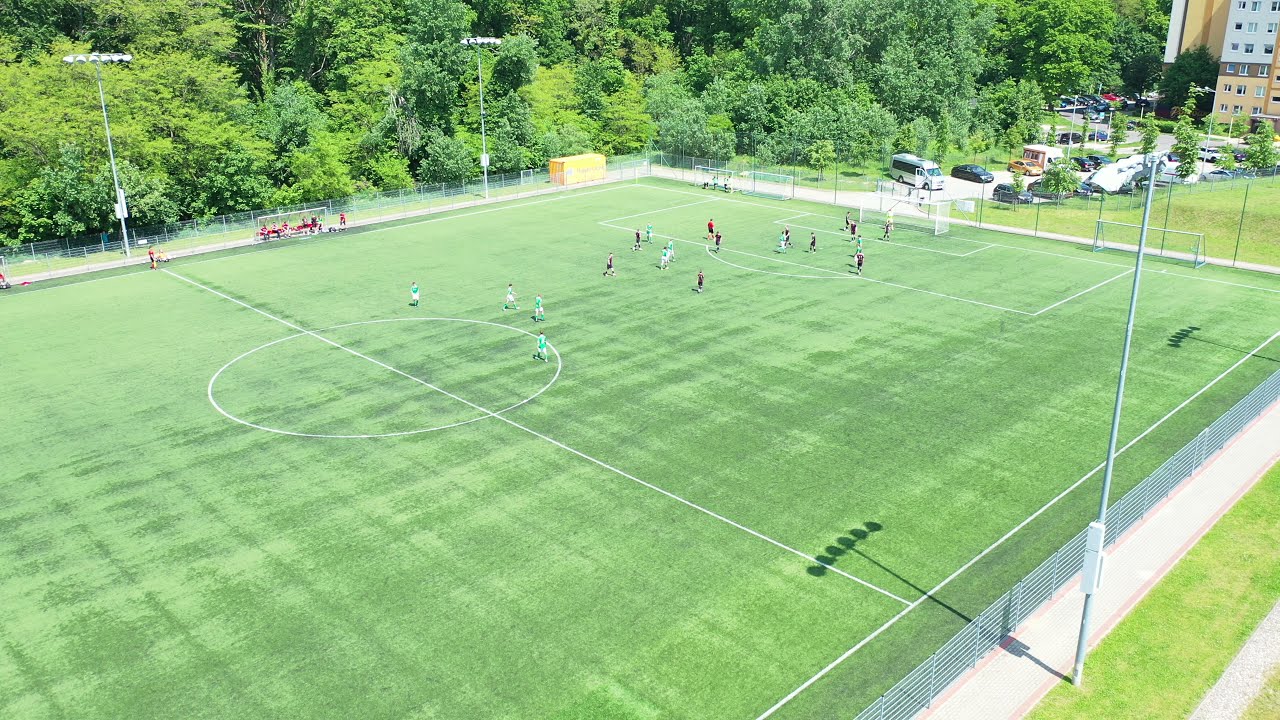The image depicts a vibrant green soccer field viewed from an elevated angle, showcasing a bustling match in progress. In the center of the field, a large white-outlined circle is bisected by a horizontal line dividing the rectangular field into two halves. The players are predominantly concentrated on the right side of the field. Two teams compete; one team is in white jerseys, while the opposing team is in red and black. Notably, another detail describes some players, particularly those on the bench, wearing red shirts with some in black and white pants. The white goal stands prominently on the far right side of the field. Surrounding the entire field is a metal fence.

Adjacent to the field, to the right side of the image, there's a parking lot populated by various vehicles, including a white van, black sedans, and a yellow sedan. This parking area is bordered by a two-story building with 21 windows arranged in a pattern of three across and seven vertically. This building, noted as either white or light brown, stands out with its distinct orange hue.

Tall outdoor lights with six individual bulbs each illuminate the field, and behind them lies a dense array of trees with varied green foliage, suggesting a subtropical environment. The upper right-hand corner of the photograph features these trees, contributing to the lush, verdant backdrop, which tapers off into the distant horizon.